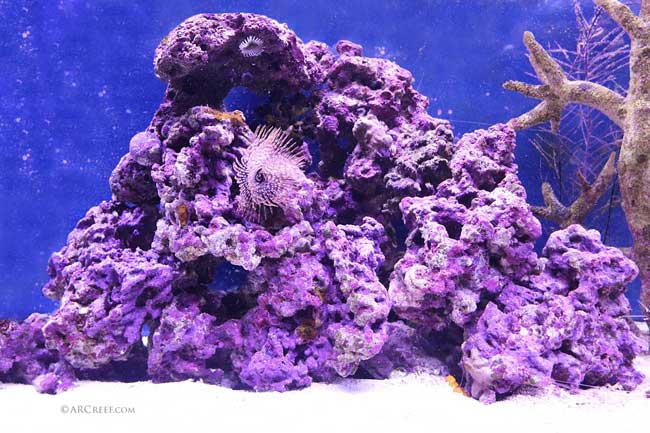In the image, we see an underwater scene featuring a vividly purple coral reef structure, characterized by numerous holes and crevices. This pyramid-shaped formation, resembling a rock with a detailed, coral reef-like appearance, dominates the foreground. The coral is dotted with small, spiky fish that appear to take refuge in its crevices. The backdrop is a deep blue sea with visible bubbles and light filtering through, hinting at relatively shallow waters. On the far right side of the image stands a contrasting aquatic plant, brown and slightly gray, with a tree branch-like structure adding intriguing variety to the scene. Notably, the bottom left corner of the image displays the text "ARC or EET.com" in gray, suggesting a watermark. This well-lit, captivating underwater photograph intricately captures the colorful and diverse marine life.